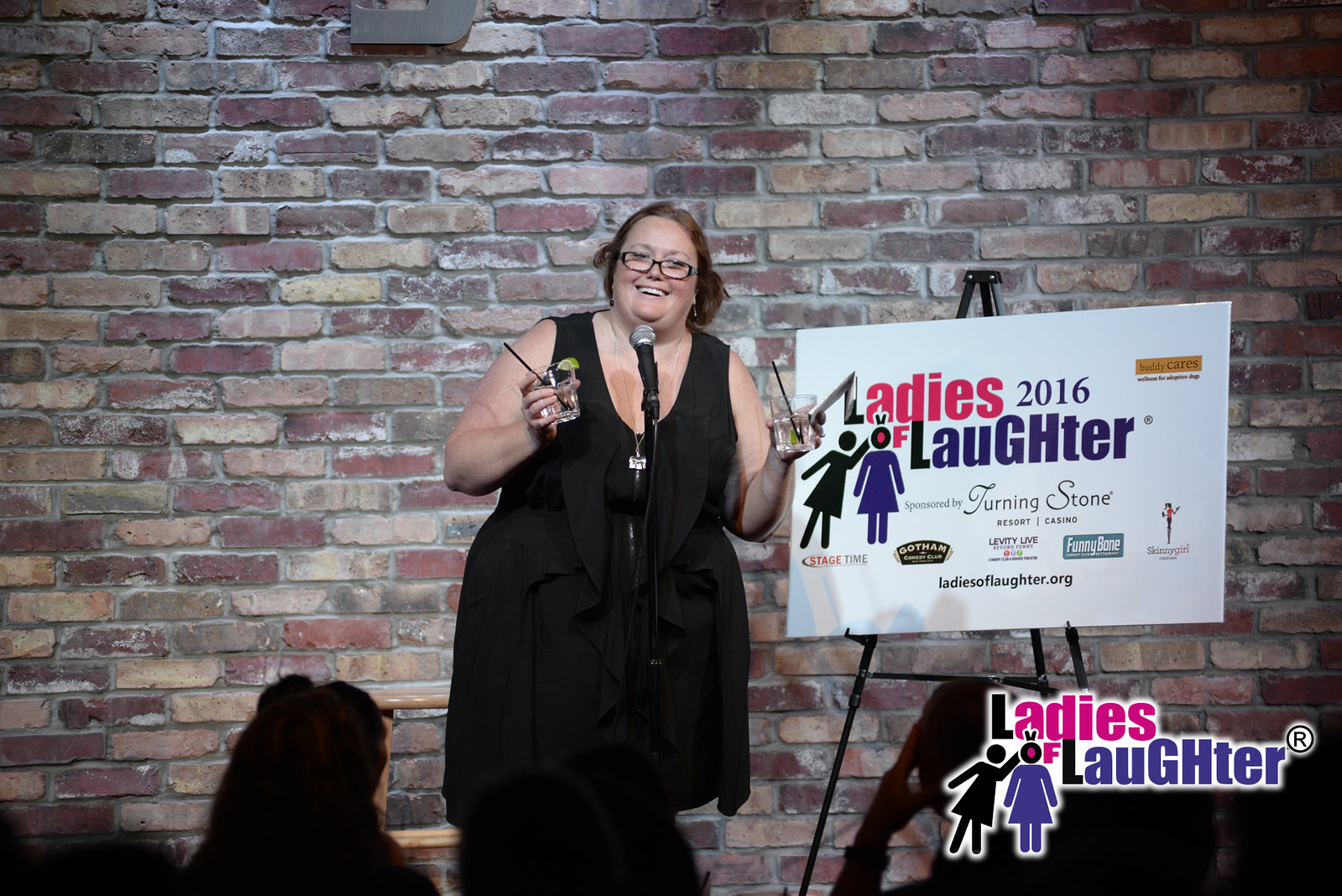A woman, dressed elegantly in a sleeveless black dress, stands confidently on stage addressing an audience. She wears glasses and has a bright, engaging smile, suggesting she is enjoying the moment. Holding a microphone on a stand with one hand, she grasps a glass containing a fancy drink in the other, complete with a stirring straw and a garnish, possibly an umbrella or a slice of lime. In her other hand, she holds a similar drink, adding to the festive atmosphere. The backdrop features an exposed brick wall, giving the setting an industrial design vibe, and is bathed in dramatic spotlighting. The heads of attentive audience members are silhouetted in the foreground, emphasizing their focus on her. To her side, a stand displays a sign that reads: “Ladies 2016 Laughter sponsored by Turning Stone. Ladiesoflaughter.org,” indicating that this event is part of a special comedy performance or gathering dedicated to showcasing female comedians.